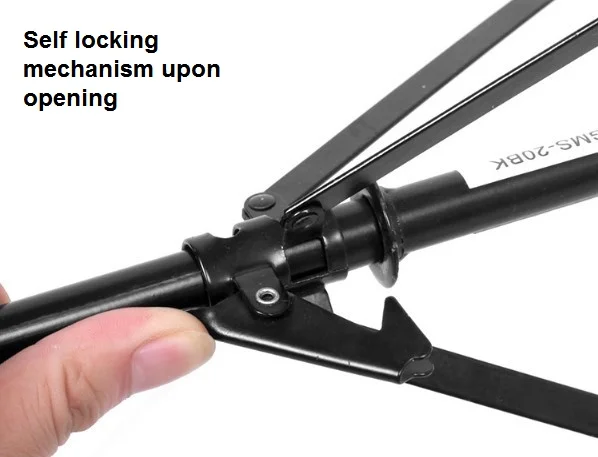The photograph depicts a glossy black metal tripod with a cylindrical central rod and three slender arms extending from it. A self-locking mechanism is highlighted in the upper left corner with the text, "self-locking mechanism upon opening." The image shows a person's thumb pressing a lever to lock the central rod in place, emphasizing the ease of operation. The product, labeled SMS-20BK, features a detailed mechanism where pushing the central rod causes three prongs to extend outward. The central focus of the image is the self-locking mechanism activated by the thumb, showcasing the functionality and design of the tripod.